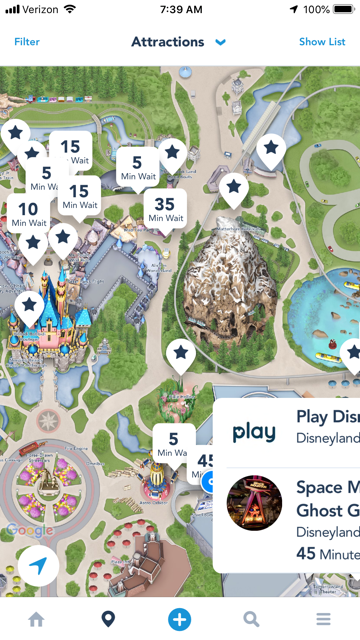This detailed caption provides a comprehensive description of a screenshot taken from a user's cell phone displaying an illustrated overhead view of Disneyland:

---

Screenshot from a cell phone displaying a detailed overhead illustrated view of Disneyland. The status bar at the top shows the user is connected to the Verizon network with full Wi-Fi and cell coverage, the time is 7:39 AM, and the battery is fully charged at 100%. The screen is filtered under "Attractions," and "Show List" is an option below the filter.

The central portion of the image presents an illustrated map of Disneyland, highlighting various attractions marked by location icons with stars. Some attractions include estimated wait times: 10 minutes, 5 minutes, 15 minutes (twice), 35 minutes, and others just feature stars without time details.

Prominent landmarks in the illustration include Cinderella's Castle, Thunder Mountain, a water feature, a grassy area, and a statue of Walt Disney and Mickey Mouse surrounded by flowers.

On the right-hand side, partially visible labels read "Play Disneyland" and cut-off text indicates "Space M…" and "Ghost G…". It's noted that an attraction named "Disneyland" has a wait time of 45 minutes.

The interface at the bottom of the screen displays icons for Home, Location, Plus, Search, and Menu. Additionally, the URL "www.microsoft.com" is shown twice at the bottom of the image.